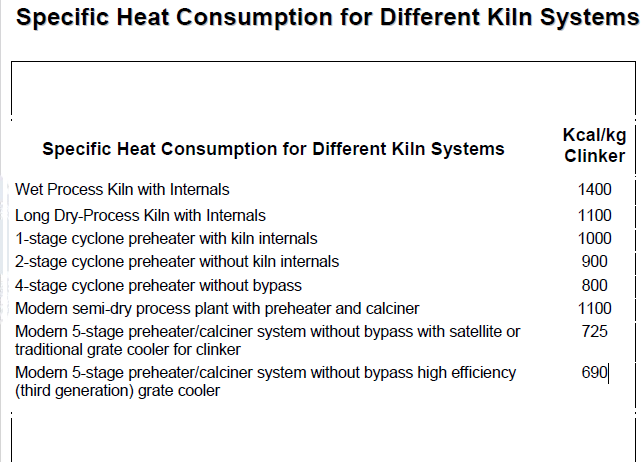The image features a printed page with the title "Specific Heat Consumption for Different Kiln Systems" at the top, rendered in black text. This title is repeated within a rectangular border, which is faded on the left and right sides and lacks a bottom line. Below the title, the left-aligned text details various kiln systems and their corresponding specific heat consumption values, measured in kilocalories per kilogram (kcal/kg), under the heading "kcal/kg Clinker" on the right side. The systems and their values are: "Wet Process Kiln with Internals" at 1400 kcal/kg, "Long Dry Process Kiln with Internals" at 1100 kcal/kg, "One Stage Cyclone Preheater with Kiln Internals" at 1000 kcal/kg, "Two-Stage Cyclone Preheater without Kiln Internals" at 900 kcal/kg, "Four-Stage Cyclone Preheater without Bypass" at 800 kcal/kg, "Modern Semi-Dry Process Plant with Preheater and Calciner" at 1100 kcal/kg, "Modern Five-Stage Preheater/Calciner System without Bypass with Satellite or Traditional Grate Cooler for Clinker" at 725 kcal/kg, and "Modern Five-Stage Preheater/Calciner System without Bypass, High Efficiency, Third-Generation Grate Cooler" at 690 kcal/kg. The entire layout is predominantly white with black text, and the delineating lines around the text are partially visible.